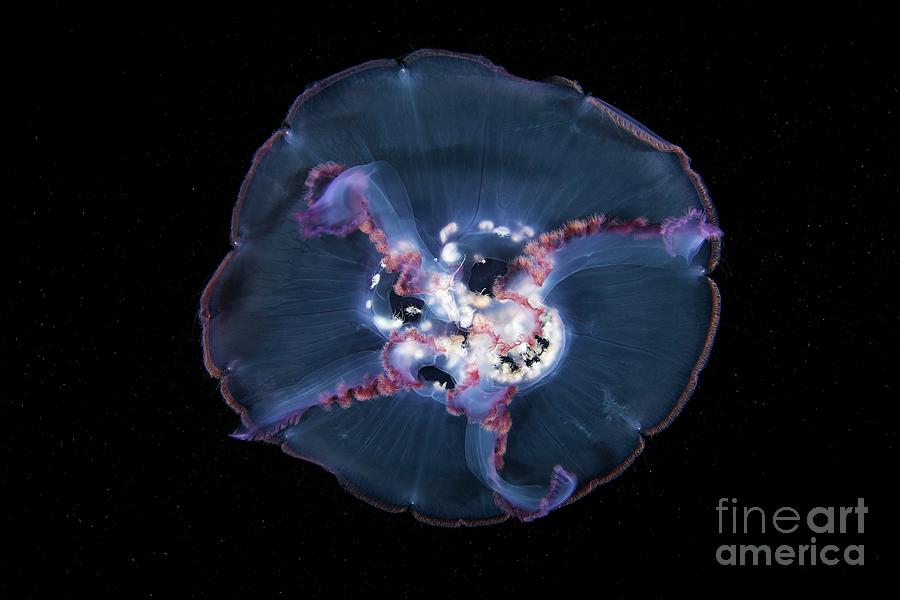The photograph features a stunning top-down view of a translucent, bluish jellyfish against an all-black background. The center of the image highlights the jellyfish's round umbrella-like body, which appears almost flower-like with petal-like formations. Its luminescent interior glows with bright white and purple hues, while delicate, hair-like tendrils extend outward. These tendrils include reddish and white clusters that add to its ethereal appearance. The jellyfish's four primary tentacles, resembling arms, stretch out from underneath its body. A subtle brownish rim traces the edge of its translucent, blue umbrella. In the bottom right corner of the photo, the inscription "Fine Art America" is visible, indicating the artwork's origin.